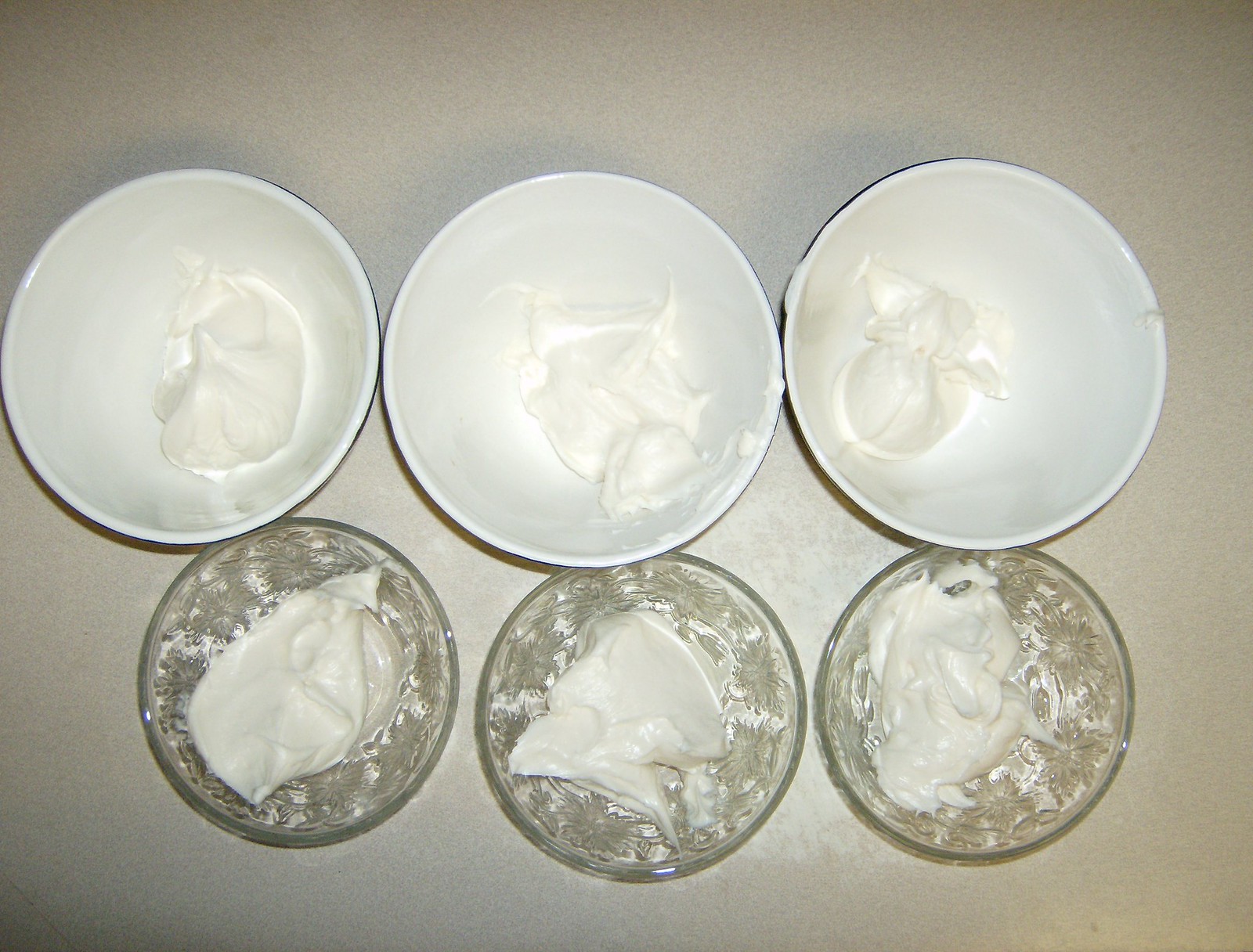In this top-down photograph, we observe six evenly spaced, white ceramic bowls arranged on a tan-brown countertop. Each bowl, seamlessly paired with a glass bowl directly in front of it, contains a rich, thick, creamy white substance. The substance within the bowls, likely a type of mayonnaise, moisturizer, or meringue, gleams under the light, adding to its smooth, gelatinous appearance. The ceramic bowls are uniform in shape and size, flaunting a classic white interior, and the glass bowls in front of them feature an elegant starburst pattern etched into the glass. The arrangement forms a coordinated layout of rich textures and creamy consistencies on a subtly contrasting background.